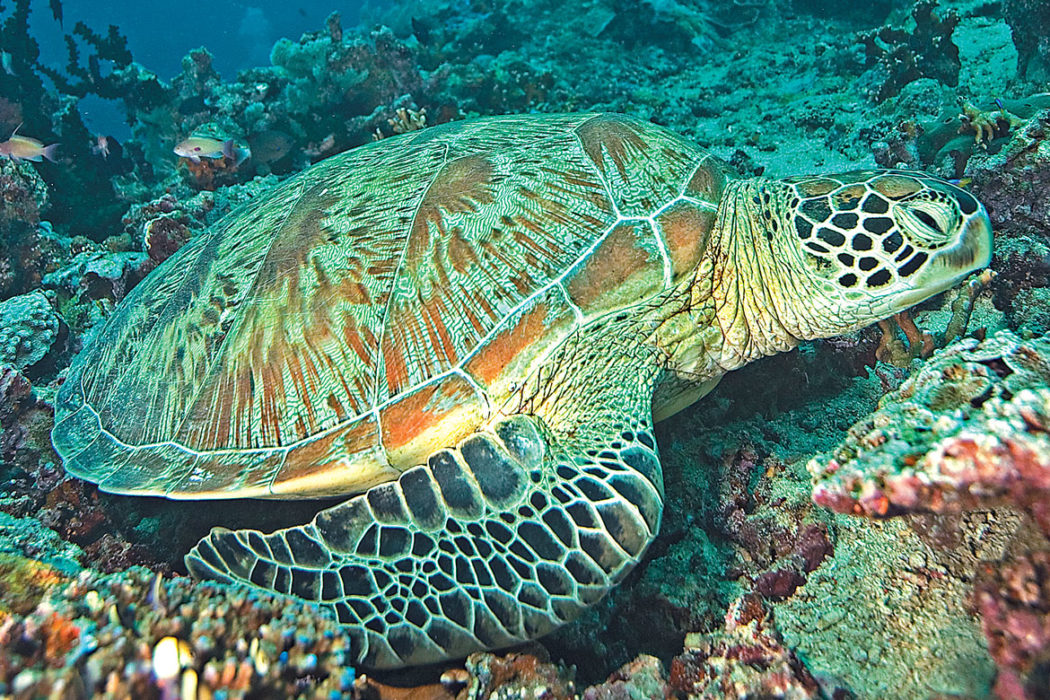In this striking underwater photograph, a large sea turtle rests serenely on a coral reef. The scene is bathed in the clear, light blue waters of the ocean, where vivid marine life thrives. The turtle, with its eyes half open, appears as if it’s taking a leisurely nap amidst this vibrant ecosystem. The turtle’s shell is a mesmerizing blend of turquoise with accents of brownish red and hints of green, intricately textured and slightly rounded. Its limbs and face are a darker, almost black hue, detailed with patches of white, adding to its majestic presence. Surrounding the turtle, the reef teems with life, including smaller fish and possibly a crab or two, all set against a backdrop of diverse coral structures that extend into the deeper, darker shades of blue ocean in the distance. The photograph captures the turtle in a moment of stillness and beauty, offering a glimpse into the tranquil yet bustling underwater world.